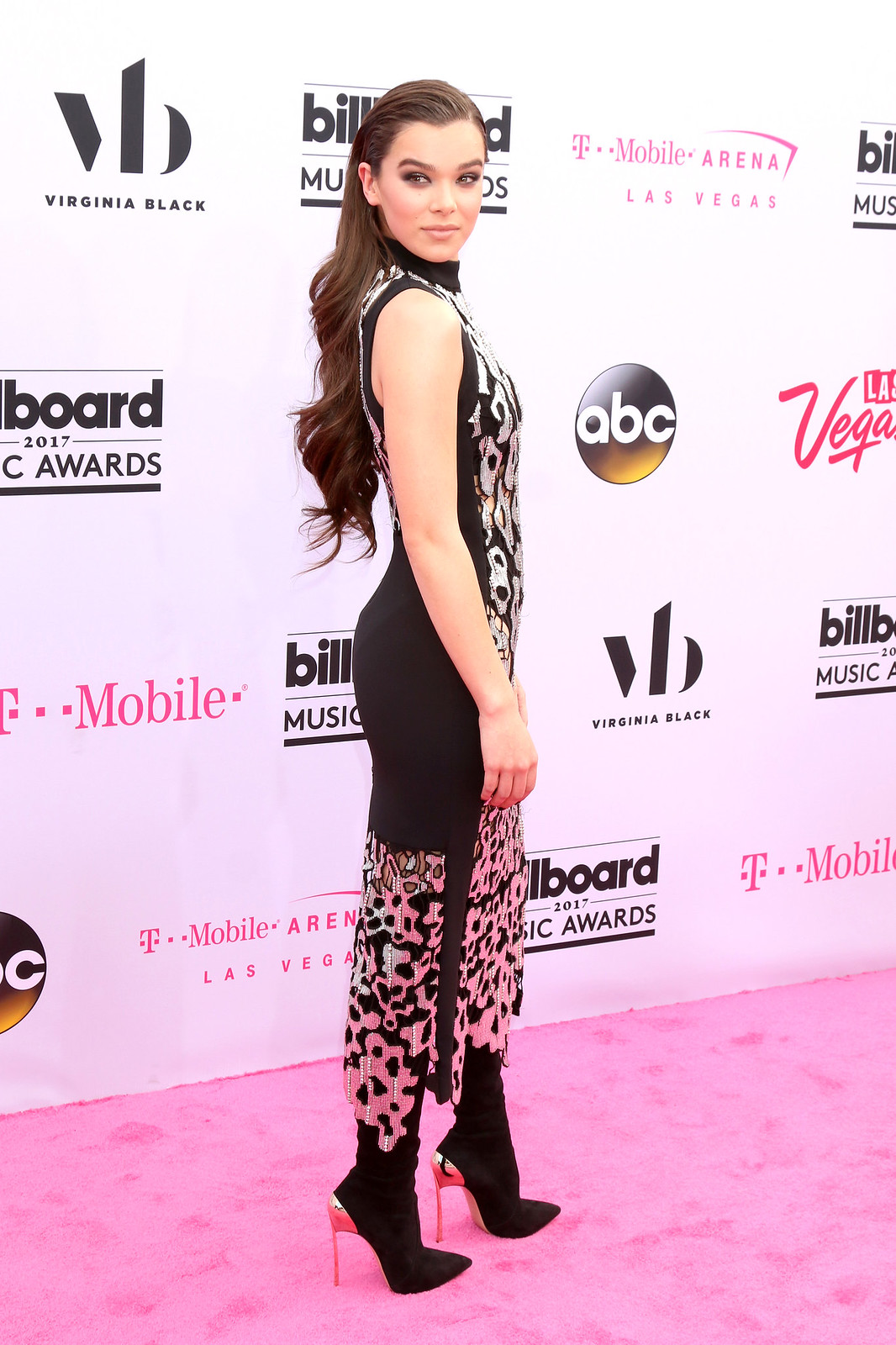This photograph captures a young woman, likely in her late teens or early twenties, posing elegantly on a pink and red carpet at the 2017 Billboard Music Awards held at the T-Mobile Arena in Las Vegas. She stands in the center of the image, which is taller than it is wide, showcasing a portrait mode composition. The backdrop features a white step-and-repeat banner adorned with various logos: Billboard Music Awards 2017, T-Mobile, Virginia Black, ABC Television Network, and Las Vegas.

The woman, of Caucasian descent, has long flowing brown hair that cascades to her mid-back with curls at the ends, and she has dark eyes accentuated with significant eye makeup. She wears a sleeveless black dress with metallic, almost animal print accents, and stylish thigh-high boots with high heels that feature striking gold spikes. She appears poised with her right arm gently hanging down, her left foot forward, and her body facing right while she looks back over her shoulder, giving a graceful and confident pose.